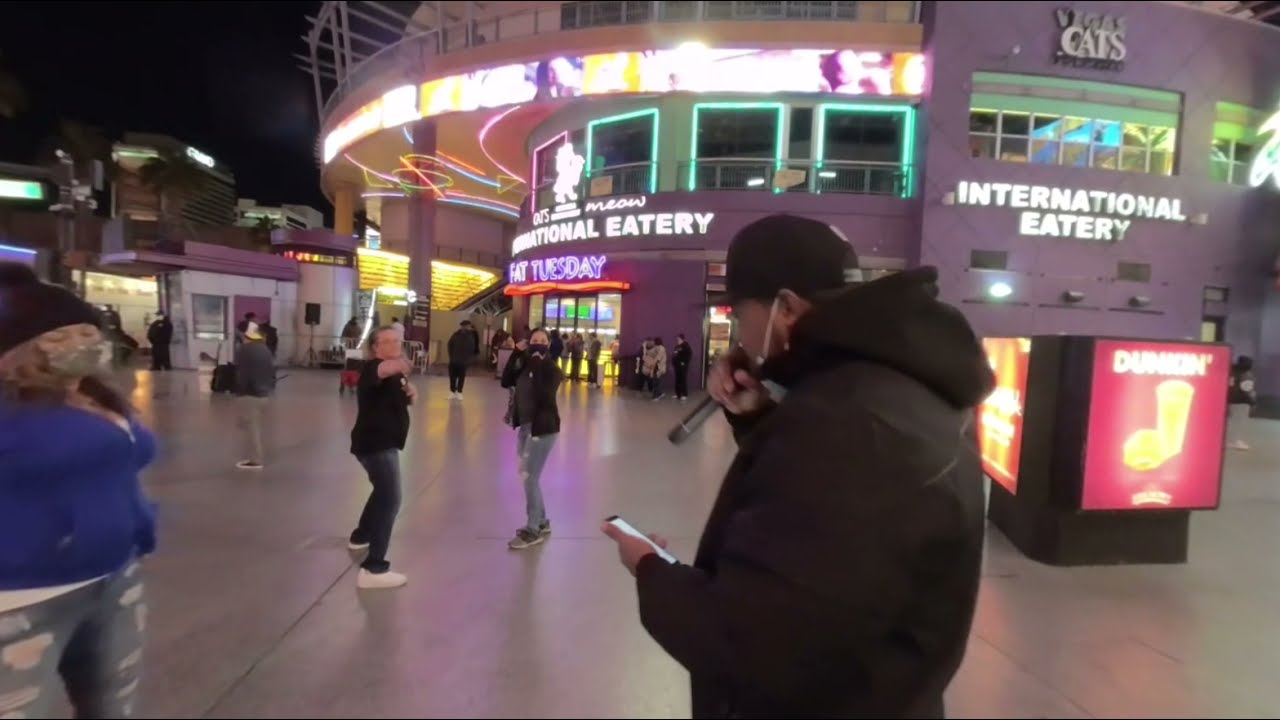The image features a bustling food court scene, potentially outdoors at night, on a surface made of large, shiny stone tiles that reflect the ambient lighting. In the foreground, a man stands slightly to the right, dressed in a black hoodie and jacket, a black baseball cap, and with a black mask pulled down to his chin. He holds a smartphone in his left hand and a microphone in his right, suggesting he might be speaking or performing. To his left, a woman wearing a black stocking cap, blue jacket, and gray jeans with holes stands looking down at him. Further in the background, two people in jeans and black shirts are seen, one pointing towards the man. The backdrop includes a rounded building with multiple illuminated signs, such as "International Eatery," "Fat Tuesday" in glowing purple letters with a red underline, and a Dunkin' Donuts ad, among others. The setting appears to be a lively gathering spot centered around various eateries.